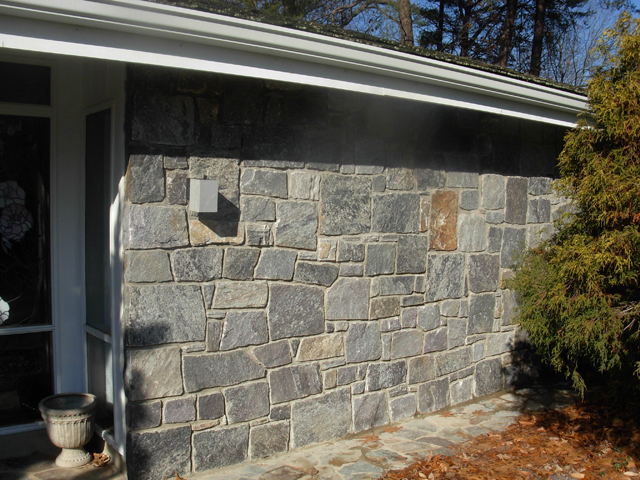This daytime photo captures the exterior of a stone-facade residence characterized by its intricate and uneven design featuring a mix of grays, browns, and tans. The partially visible asphalt roof is accompanied by white gutters, and the sun's reflection highlights the detailed stonework. To the right of the image stands a large evergreen tree, adding a touch of vibrant green against the building. The left side of the image reveals a possible front or side entry, marked by a white-trimmed glass door and a floor-to-ceiling glass window. Below the entry, an empty cement planter sits on a stone sidewalk that borders the residence. Additional details include brown leaves scattered on the ground, a small gray rectangular box on the wall that could be a sconce or power source, and a white light fixture. The background showcases a blue sky with green trees, contributing to the serene and picturesque atmosphere.